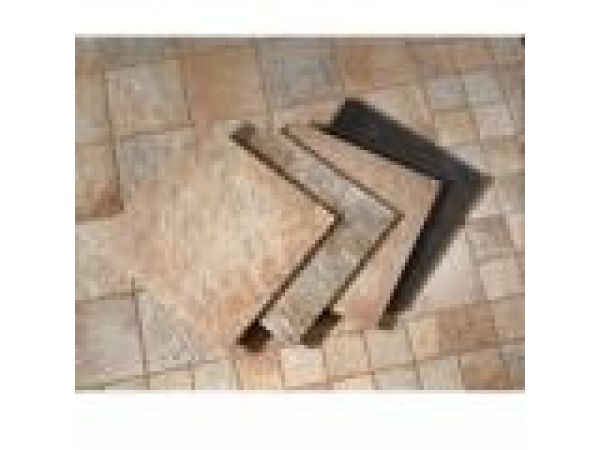This image captures a horizontal, rectangular scene focused on a tiled floor, possibly from a kitchen or basement. The background consists of various tiles in multiple sizes, with larger tiles on the left and smaller, intricate patterns on the right, creating a mosaic effect. The overall palette includes shades of brown, tan, and gray, giving the floor a harmonious yet varied appearance. Overlaid on this floor are four larger, staggered tiles, each distinct in color—ranging from light brown to dark gray. Despite the pixelation and dated quality of the image, it's clear these tiles have serrated edges due to the resolution. The arrangement seems deliberate, perhaps meant to display different tile samples.